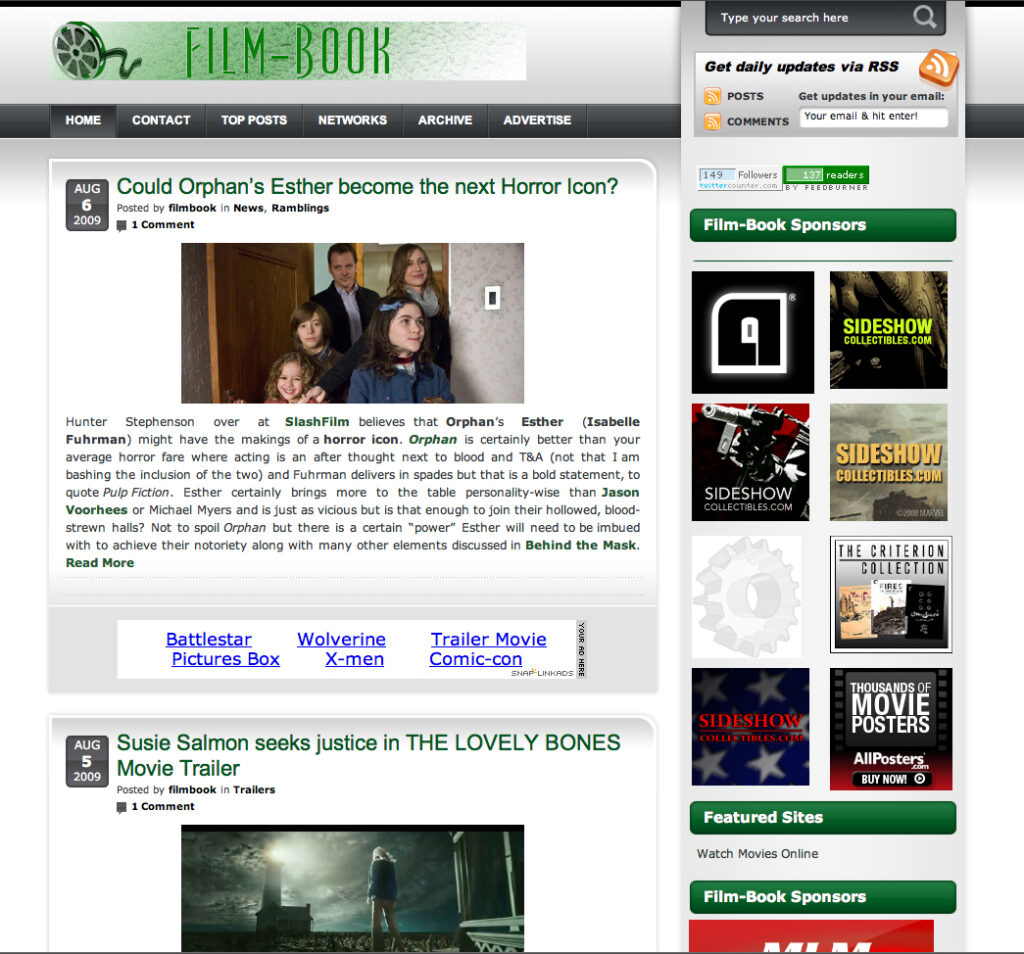This is a screenshot of a webpage from the film-book website, featuring a sleek black navigation bar at the top with white text displaying options such as Home, Contact, Top Posts, Networks, Archive, and Advertise. Below this, the headline reads, "Could Orphan’s Esther Become the Next Horror Icon?" dated August 6, 2009. The article discusses Hunter Stephan’s view from Slash Films, suggesting that Esther, portrayed by Isabel Fuhrman in the film "Orphan," has the potential to become a horror icon. It praises the movie for its superior quality compared to typical horror films, highlighting Fuhrman's exceptional performance. The writing delves into a bold comparison, quoting "Pulp Fiction," claiming Esther brings more personality to the table than established characters like Jason Voorhees or Michael Myers, despite matching their levels of brutality. However, it also notes that for Esther to join the ranks of such iconic figures, she would need to possess a certain power to achieve their legendary status.